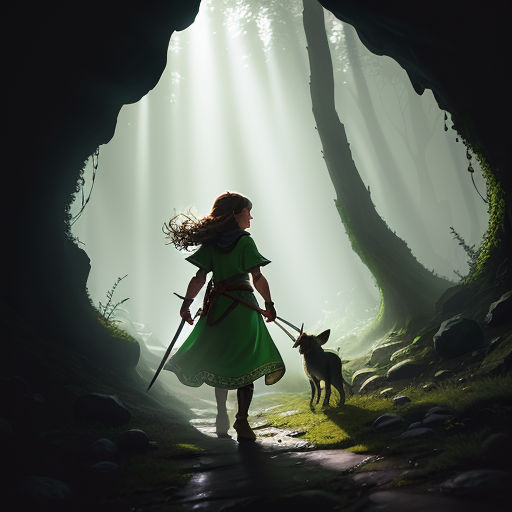The illustration depicts a young girl, dressed in a short-sleeved green dress, with long flowing brown hair, walking her small brown dog on a leash that is wrapped around her waist. In her left hand, she holds a stick, possibly a staff or a walking stick. The environment suggests she's emerging from a tunnel or a cave into a sunlit forest. The scene is framed by grayish-black walls with moss growing at the entrance, creating a natural tunnel of light through the tall tree trunks. The narrow, brown-hued path is bordered by moss, ferns, short grasses, small pebbles, and larger rocks. Sunlight beams down from the canopy above, casting light on the serene woodland setting. The overall impression is one of an adventurous journey through a mystical, forested landscape.